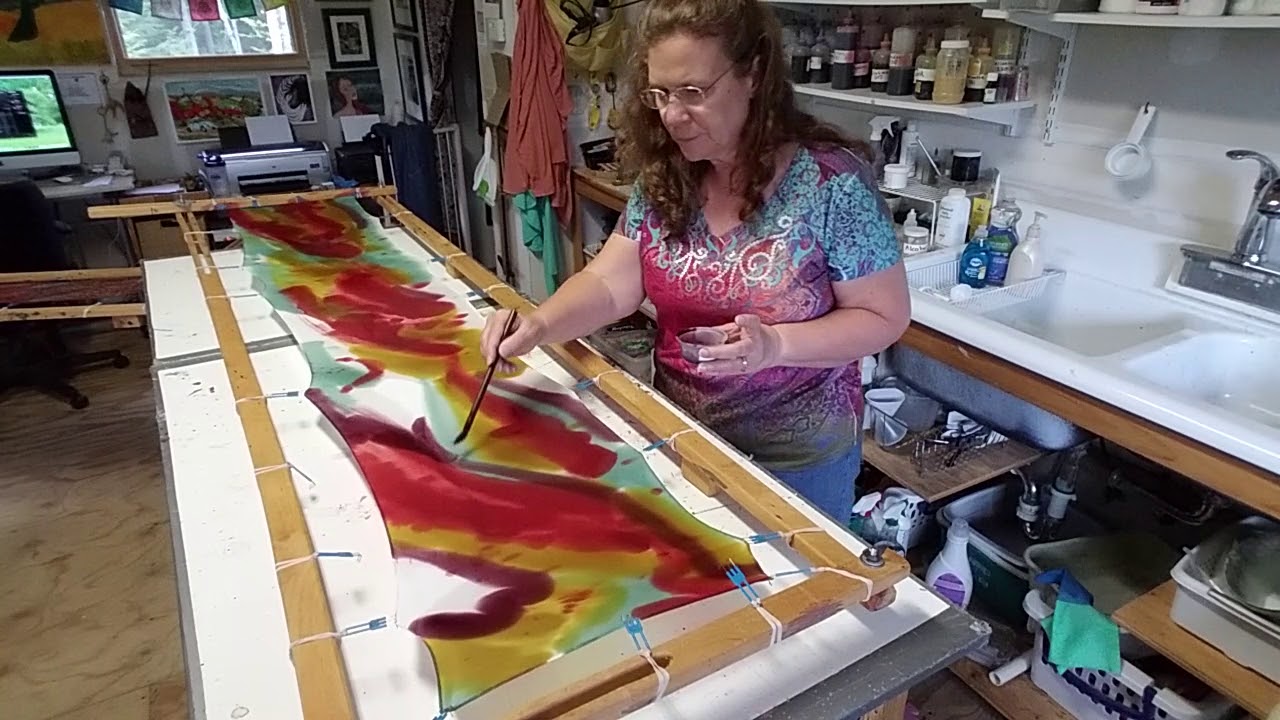In the image, a female artist, possibly around 50 years old, is immersed in her creative process within a well-organized art studio. She stands at a long countertop table, diligently painting on a large piece of fabric stretched over a wooden frame. Her detailed attention is evident as she skillfully uses a thin black brush held in her right hand, while her left hand holds a tiny cup of paint. The fabric, adorned with a blend of reds, yellows, and greens, displays an abstract design with colors melting toward the side.

The woman has curly brown hair and wears glasses, along with a vibrant, multicolored t-shirt dominated by blue and reddish hues. Behind her, a spotless white sink is visible, surrounded by shelves loaded with various art supplies. To her left, there's a computer and a printer on the table, beneath a window garnished with hanging flags. Several framed photos are also arrayed next to the window. The back wall of the studio features hooks holding an assortment of blouses and aprons, emphasizing the space's functional and creative atmosphere. The room is bathed in natural light, further highlighting the artist's focused expression and her ongoing masterpiece.